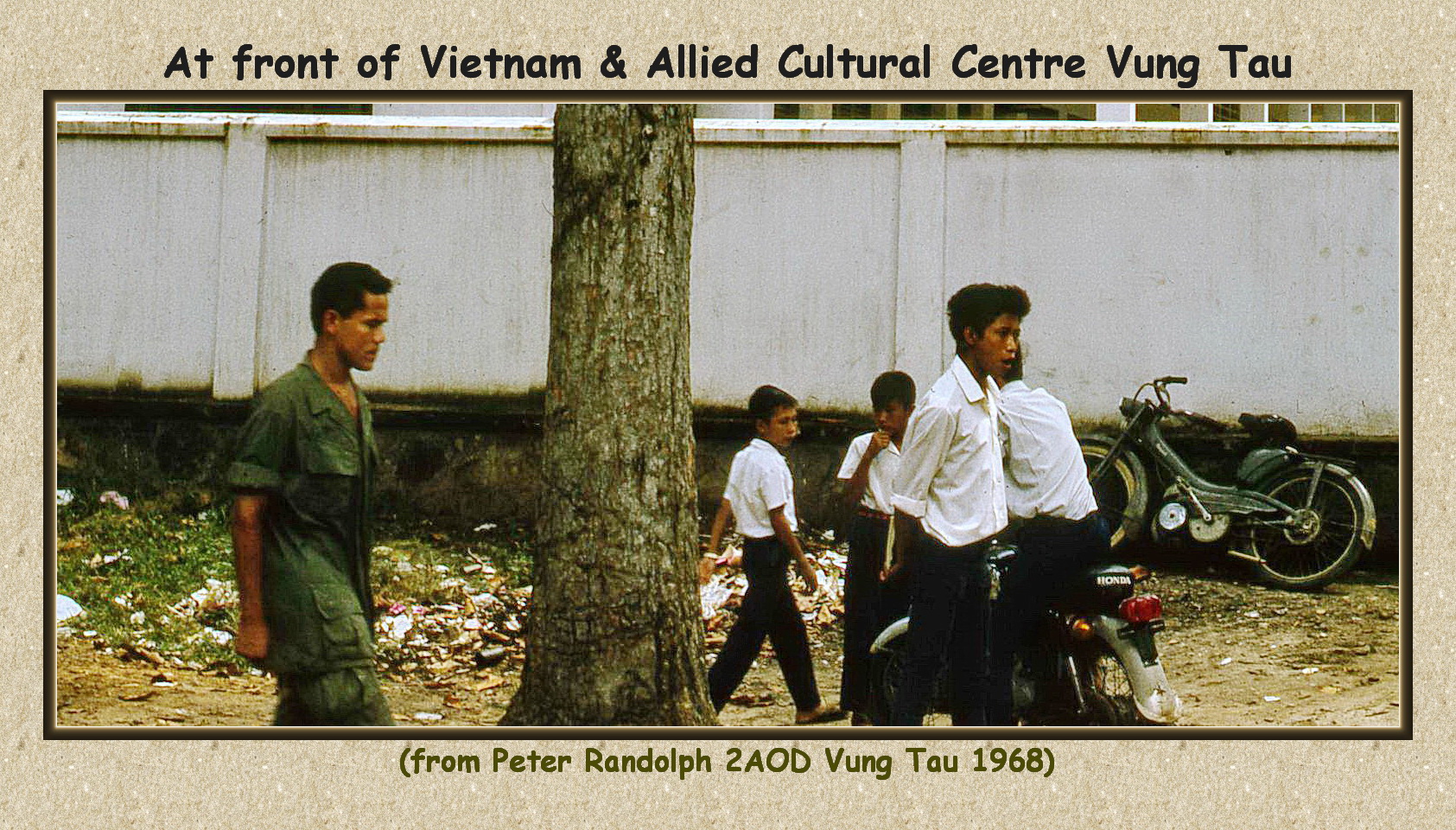The image features an old, somewhat faded, outdoor color photograph framed by a tan border with a dark brown inner border. The tan border contains the inscription in black font at the top, "At Front of Vietnam and Allied Cultural Center Vung Tau," and at the bottom in green text, "From Peter Randolph to AOD, Vung Tau, 1968." The center of the photograph shows a scene with a white painted wall in the far background, against which an old motorcycle leans. Prominently displayed in the center is a tree trunk. On the right side of the tree trunk are four young males, all dressed in white short-sleeve button-up shirts and black pants, with one of them seated on another motorcycle. To the left of the tree trunk stands a man in green military fatigues. The scene captures a moment in time at the Vietnam and Allied Cultural Center in Vung Tau.